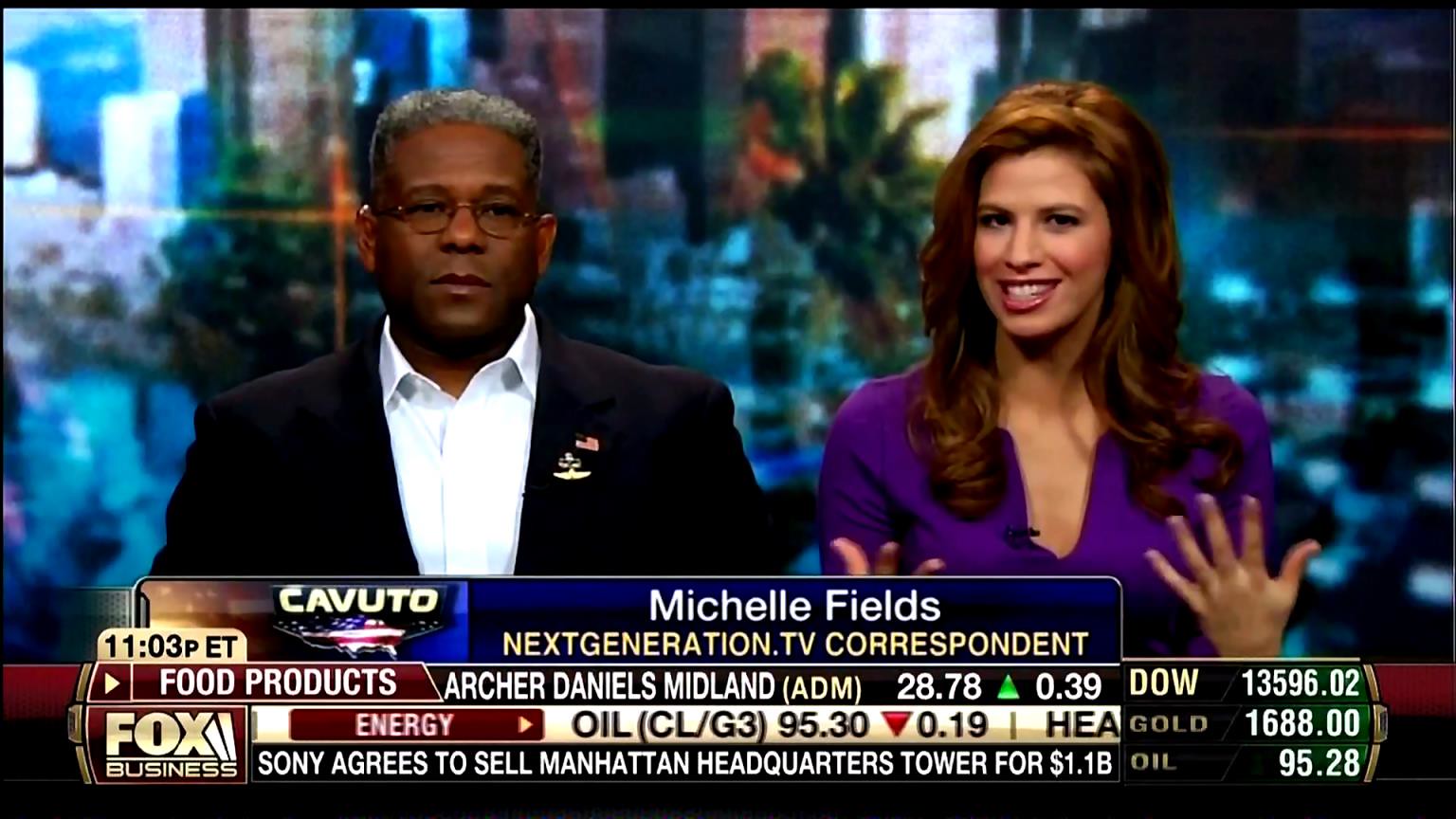This screenshot from a televised newscast features an African American man, dressed in a black suit jacket over a white shirt, accented with an American flag lapel pin and another pin resembling wings. He is seated next to a Caucasian woman with long brown hair, wearing a purple dress. The man, wearing eyeglasses, is not smiling, while the woman has her hands raised mid-conversation and is smiling. The backdrop displays a cityscape.

Below them, the text reads "Cavuto," accompanied by an American flag, and "Michelle Fields, Next-Generation TV Correspondent." Additional text overlays indicate the time as 11:03 p.m. Eastern Time and provide market updates: Archer Daniels Midland (ADM) at 28.78, up 0.39; Dow at 13596.02; Gold at 1688.00; and Oil at 95.28, down 0.19. The Fox Business logo is in the bottom left corner, and a ticker announces, "Sony agrees to sell Manhattan headquarters tower for 1.1 billion dollars."